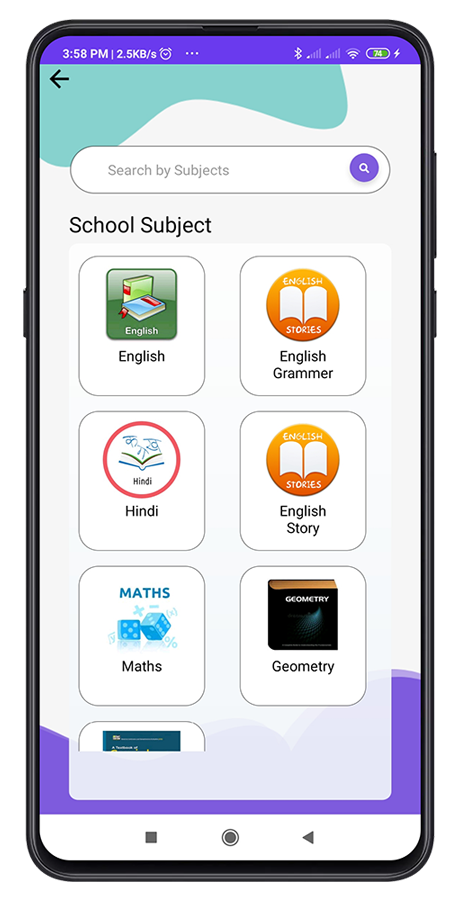This image shows a detailed screenshot of a mobile app page, depicted within the frame of a stylized cell phone. The cell phone graphic features a sleek, rounded black bezel with curved corners. On the left side of the phone, there is a single protruding button, while the right side hosts two buttons, with the upper one being taller.

At the screen's top, a purple header spans from left to right, displaying various icons and text in white. It reads "3.58pm" followed by "2.5 kilobytes per second." To the right of this, there's a white alarm clock icon, followed by three horizontally arranged white dots. Further along the top-right corner, a series of small icons are aligned: a Bluetooth logo, two identical mobile signal bars (only the first is filled in with white), a WiFi icon with three out of four bars filled, and a rounded battery icon marked "74" in white, indicating a 74% charge within a green rectangle. Adjacent to the battery icon, a small white lightning bolt signifies that the phone is charging.

Beneath the header, the main content of the page is displayed against a largely light gray background, accented by a teal splotch in the top-left corner and a purple splotch in the bottom-center. At the top center, there is a white search bar with a dark gray border, containing light gray text that reads, "search by subjects." On the far right side of the search bar, a purple circle houses a white magnifying glass icon.

Directly below the search bar, the text "school subject" appears in black on the left side of the page. Beneath this heading, a translucent white rectangle features a series of icons representing different subjects. These icons are labeled: "English," "English grammar," "Hindi," "English story," "Maths," "Geometry," and an obscured subject icon. Each labeled icon includes a corresponding image, adding a visual element to the otherwise text-centric display.